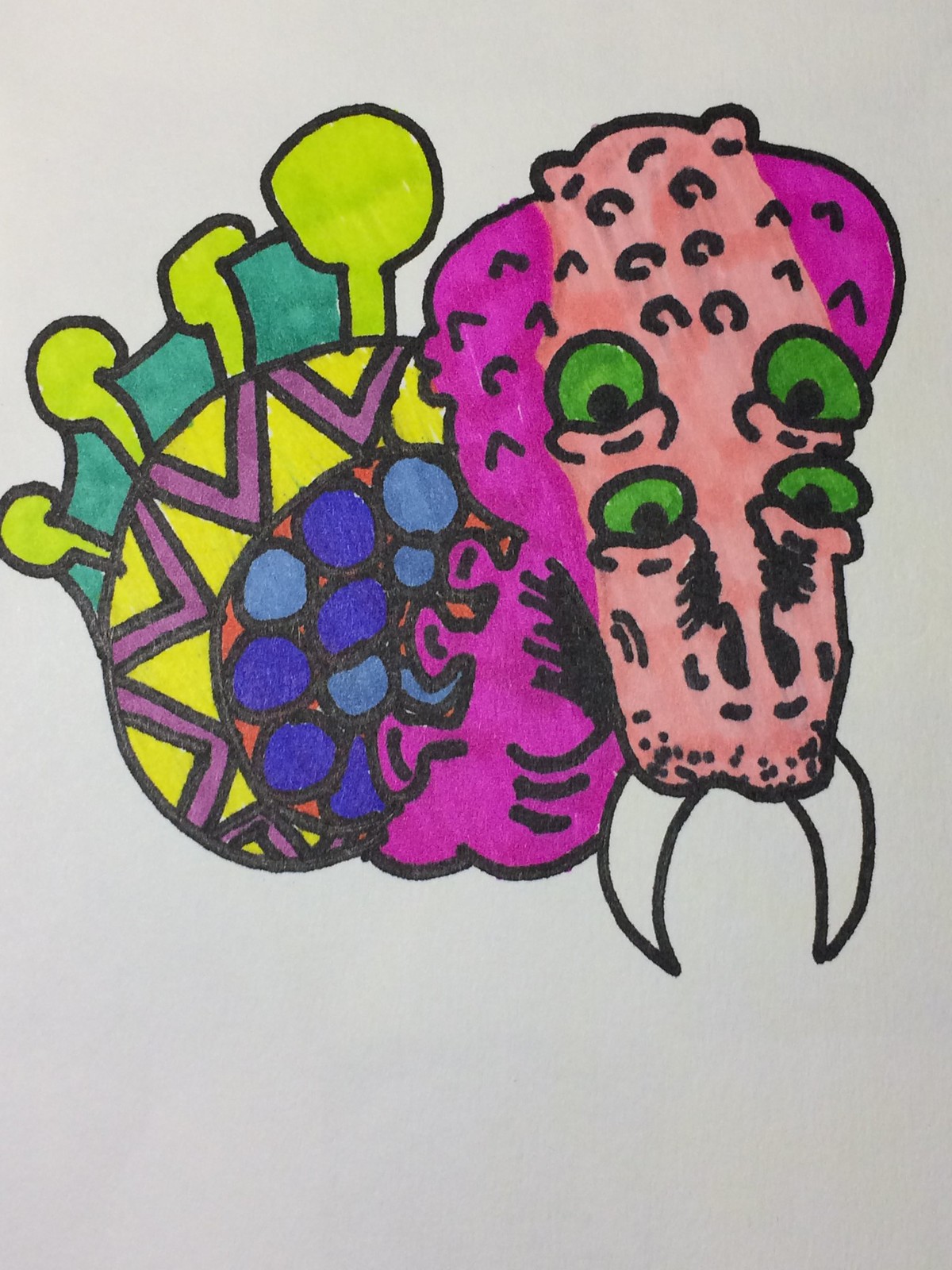This vibrant, detailed marker drawing on gray paper portrays a fantastical creature with an elongated, dragon-like head resembling both a dragon and an alligator. The head, adorned with peach and bright pink hues accented by black markings, features four vivid green eyes with black pupils. Two prominent, walrus-like white tusks trim the mouth area in black. The head transitions into a purple neck with textured black half-circles and Frankenstein-like knobs on the sides. The creature's back is decorated with blue circles of varying shades, outlined in black, and transitions into a yellow tail section adorned with purple V-patterns. Completing the vivid design, a fin-like structure in alternating dark and bright green, along with chartreuse sections, crowns the tail, adding a whimsical touch to the overall creature.